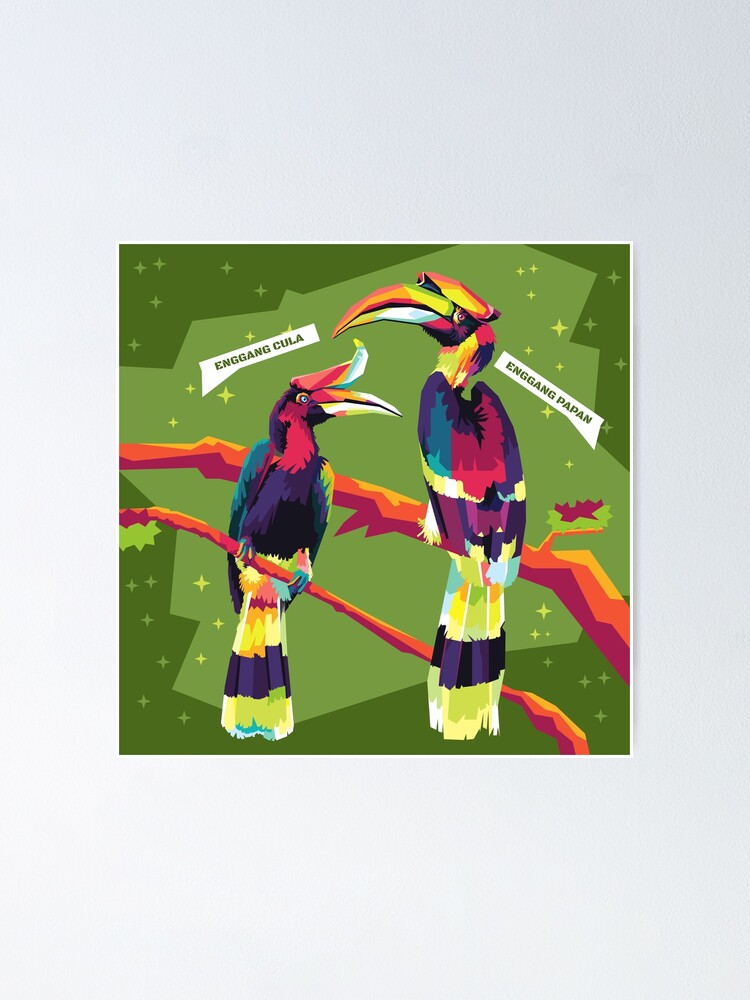This detailed illustration depicts a pair of hornbill birds named Engangkula and Engangpapan, perched on branches and facing each other within a vibrant setting. Engangkula, positioned on the left, is slightly smaller and looks forward, while Engangpapan, on the right, shows its back view. The birds exhibit an array of multicolored feathers—including shades of blue, white, yellow, green, dark blue or black, orange, purple, fuchsia, and pink—and possess an intriguing feather on their head resembling a third beak. They are portrayed in a stylized, somewhat cartoonish manner, with geometric shapes defining their beaks and heads. The branches they sit on are thin and colored in gradients of dark purple, orange, and yellow. The background features a dynamic transition from dark green on the edges to lighter green in the center, adorned with small, cross-like star formations in yellow and green. The artwork’s abstract and colorful design, combined with the birds’ expressive postures, gives it a lively and whimsical character.